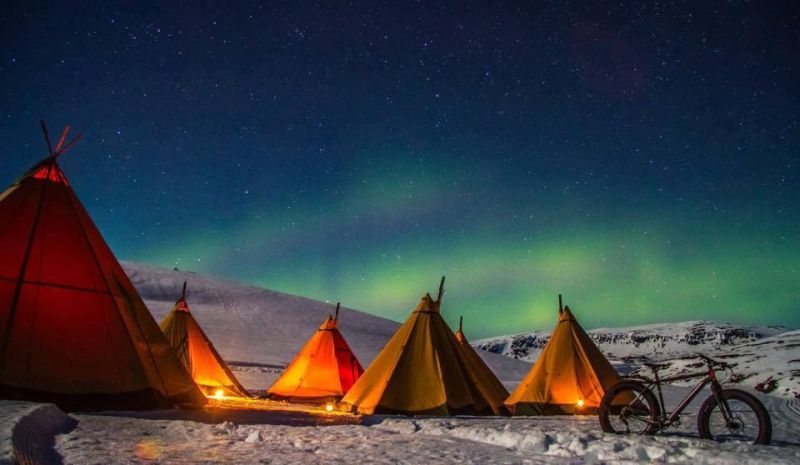The image depicts a snowy campsite at night, situated possibly in the Arctic, Antarctica, or Alaska. Several orange tents, resembling teepees, are arranged on the snowy terrain, illuminated by lights that give them a warm glow against the wintry landscape. A bicycle is parked amidst the snow near the tents. Above this scene stretches a dark navy blue sky, teeming with white stars, transitioning into a mesmerizing display of the Aurora Borealis with its green and yellow hues shimmering across the horizon. The contrasting colors of the illuminated tents and the ethereal sky create a stunning and tranquil nighttime scene.